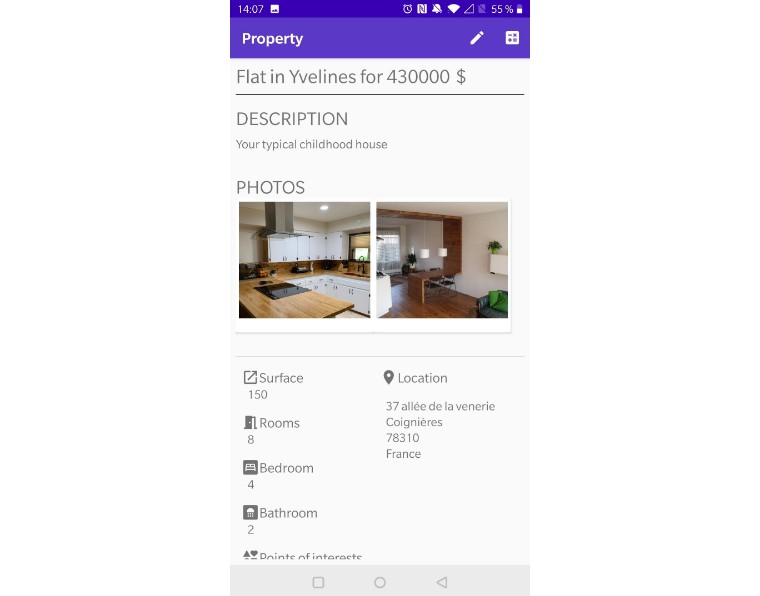Caption: 

The image showcases a property listing on a mobile app with the title "Property" and labeled as a "Flat in Yvelines" priced at €430,000. The listing describes it as a "typical childhood house" and includes two detailed photos of the interior. 

The first photo captures the kitchen, which features a stylish aesthetic with wooden countertops encompassing all sides and complemented by pristine white cabinets. The second photo highlights the living room, which intriguingly incorporates a unique dining area design. This dining table is not a traditional standalone piece; instead, it is crafted from a wooden surface that extends the length of the wall, descends from the ceiling, makes a right-angle turn at the wall, and continues down to the ground, effectively forming a functional table.

Additional information provided states a total surface area of 150 square meters, with eight rooms in total, including four bedrooms and two bathrooms. The property is located in France, with further details listed as "points of interest" though the specifics are cut off in the image.